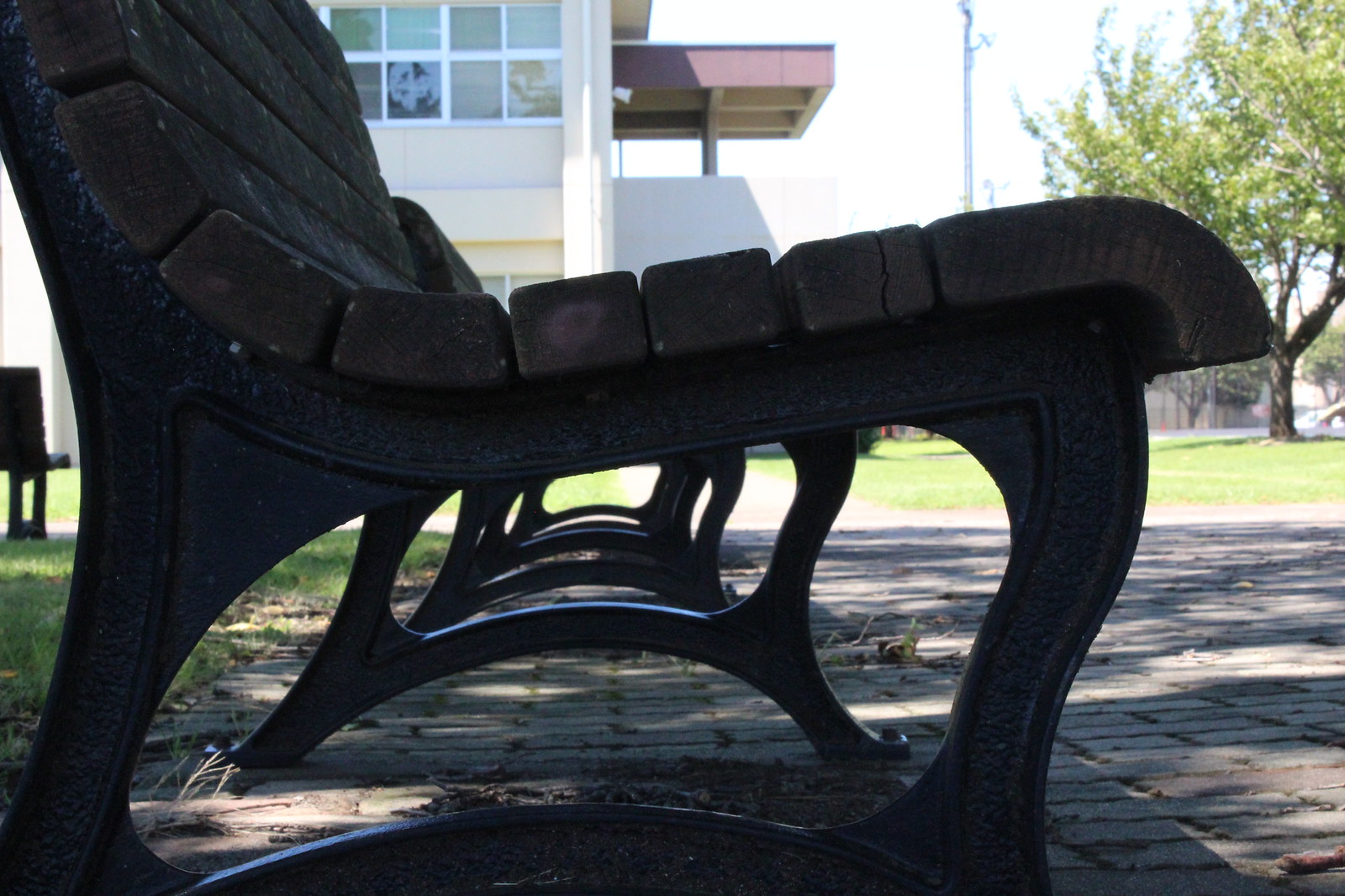This image captures an outdoor scene bathed in bright sunlight, showcasing a grassy area with a cobblestone or brick walkway. In the foreground, positioned about a foot off the ground, the camera peers directly through the base of several weathered benches, which feature steel legs and dark wooden seats. To the right, a tree provides partial shade, while in the background, a building with a distinctive purple-bordered, detached roof or awning adds an architectural element. The overall setting suggests a park or a similar outdoor seating area, giving off a serene and slightly aged aesthetic.